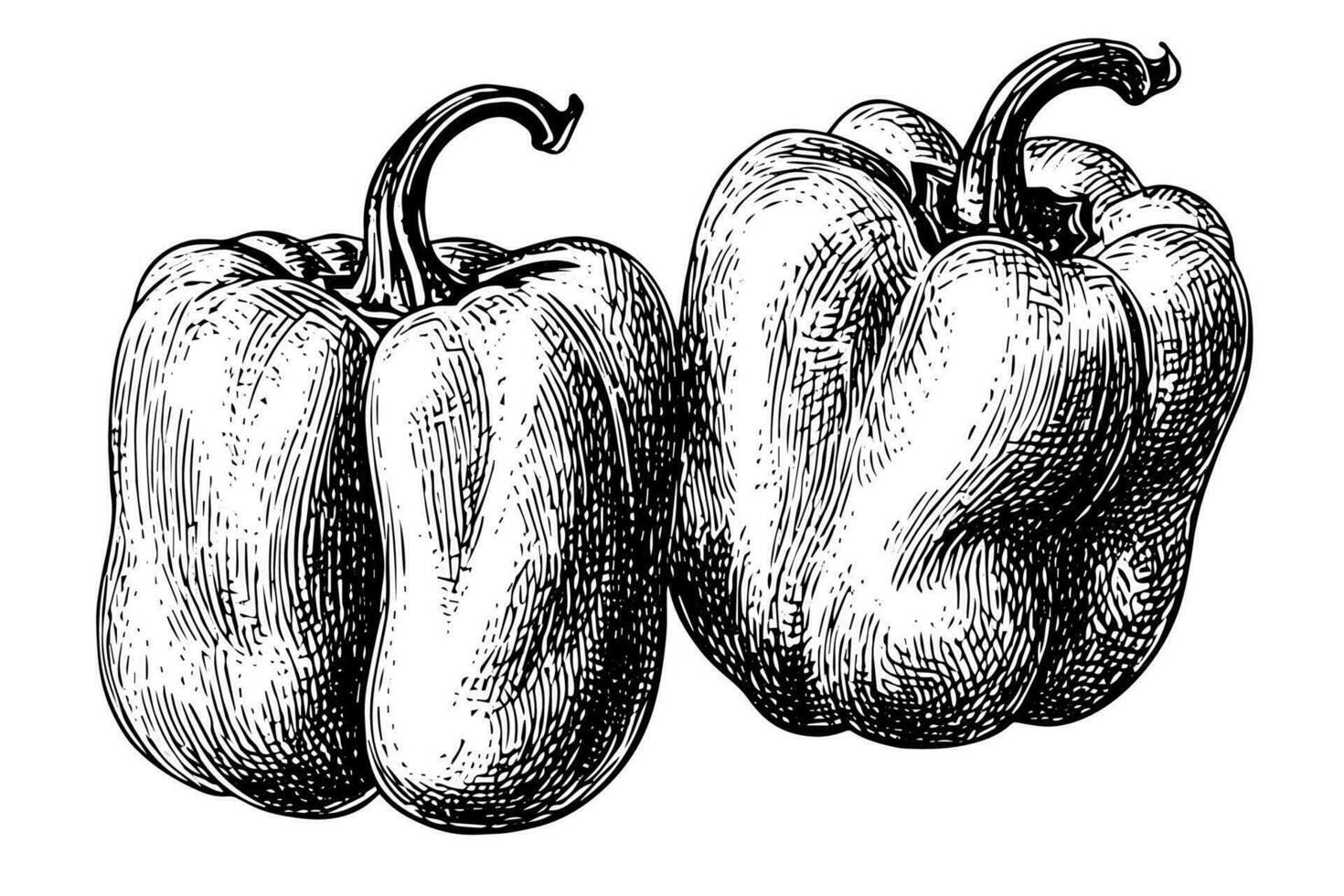This image is a highly detailed, black and white, semi-realistic ink drawing of two bell peppers set against a stark white background. The illustration showcases extensive cross-hatching and shading, enhancing the depth and dimension of the peppers, mimicking the effects of light and shadow. Depicted from left to right, the pepper on the left is slightly larger and appears undamaged, while the one on the right has a dented appearance. Each pepper's characteristic shape is meticulously rendered, from their rounded bottoms segmented into several sections, to the large bent stems culminating in pronounced, pointed tops. This detailed artwork, reminiscent of a cookbook illustration, captures the peppers in their raw, uncut state, perfect for culinary uses like bell peppers and beef or an Italian chopped sandwich.